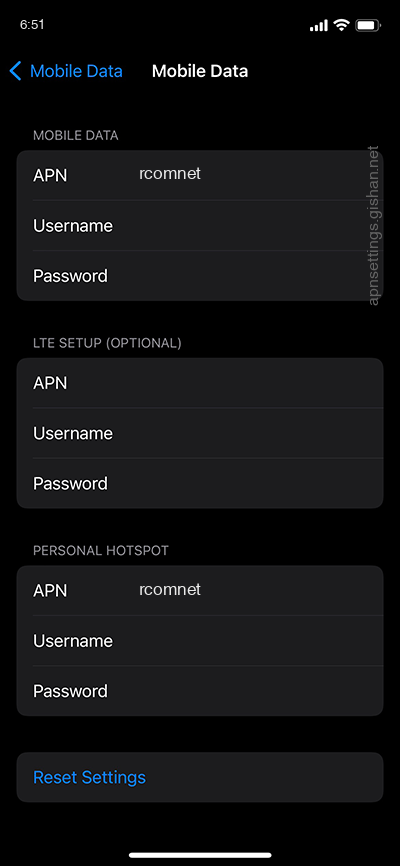Screenshot of a mobile phone with a black background. At the top left, the time is displayed in white text as "2:25". On the top right, icons show the cell signal, Wi-Fi signal, and battery status. Below, a blue arrow pointing left is followed by "Mobile data" in blue text, with "M" and "D" capitalized. In the center of the screen, "Mobile Data" is again displayed in white text with both "M" and "D" capitalized.

Further down, the text "Mobile Data" is accompanied by a lighter black rectangle with rounded corners, containing "APN" in capital letters and "RCOMNET" in uppercase text. Following this are fields for "Username" and "Password". Below this, the heading "LTE Setup (optional)" is displayed, along with fields for "APN," "Username," and "Password".

The section titled "Personal Hotspot" also displays "APN" with "RCOMNET" in uppercase, followed by "Username" and "Password". At the bottom of the screen is a lighter black banner with "Reset Settings" in bright blue text, with the letters "R" and "S" capitalized. Lastly, a thin white line is centered at the bottom of the screen.